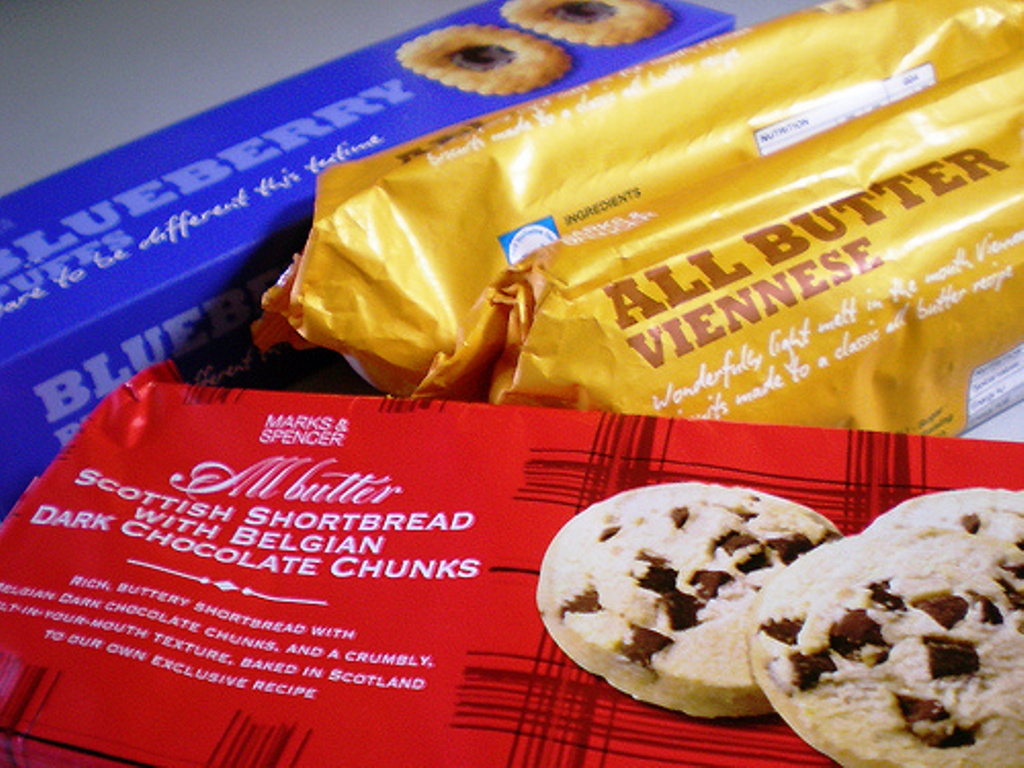The image depicts a variety of cookie packages arranged on a surface. In the far back, there is a blue package labeled "Blueberry Puffs," featuring a picture of rectangular cookies with a blueberry filling. In the middle, two packages wrapped in yellow foil are identified as "All Butter Viennese." The front package is red, labeled "M Butter Scottish Shortbread with Belgian Dark Chocolate Chunks," which includes a description saying, "rich, buttery shortbread with dark chocolate chunks and a crumbly texture." Each package features visual depictions of the cookies inside, illustrating the distinct types of treats for each type of packaging: blueberry-filled cookies, Viennese butter cookies, and chocolate chunk shortbread.